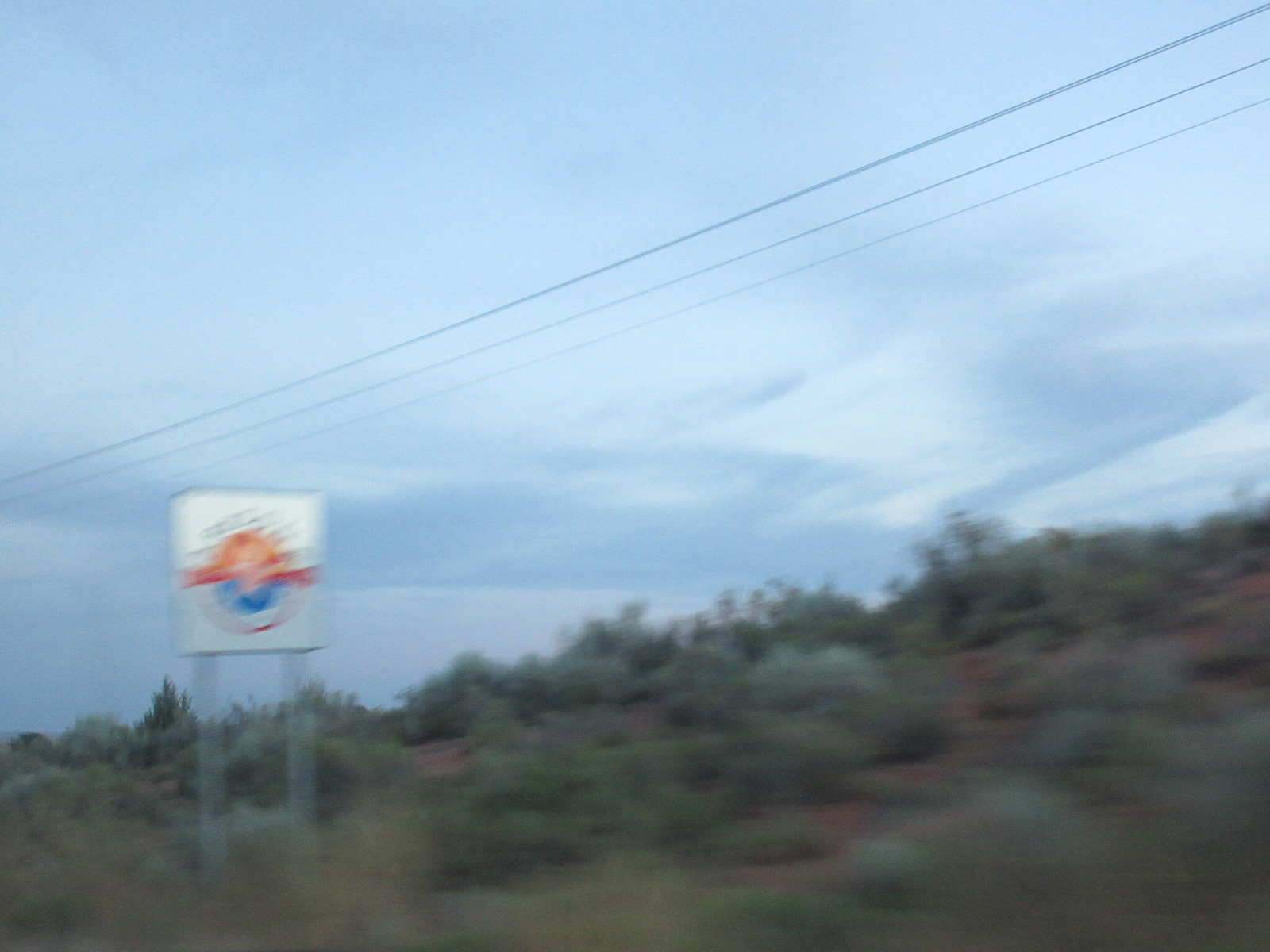This photograph captures a scenic hillside adorned with a mix of scrub, bushy plants, and scattered small trees. Stretching diagonally from the lower left to the upper right is a solitary power line, subtly intersecting the landscape. Alongside a road, possibly a highway or interstate, an out-of-focus sign stands, hinting at an upcoming business - likely a gas station or restaurant, although its details remain indistinct. The overall composition juxtaposes natural elements against minimal human infrastructure, evoking a tranquil yet transient roadside atmosphere.